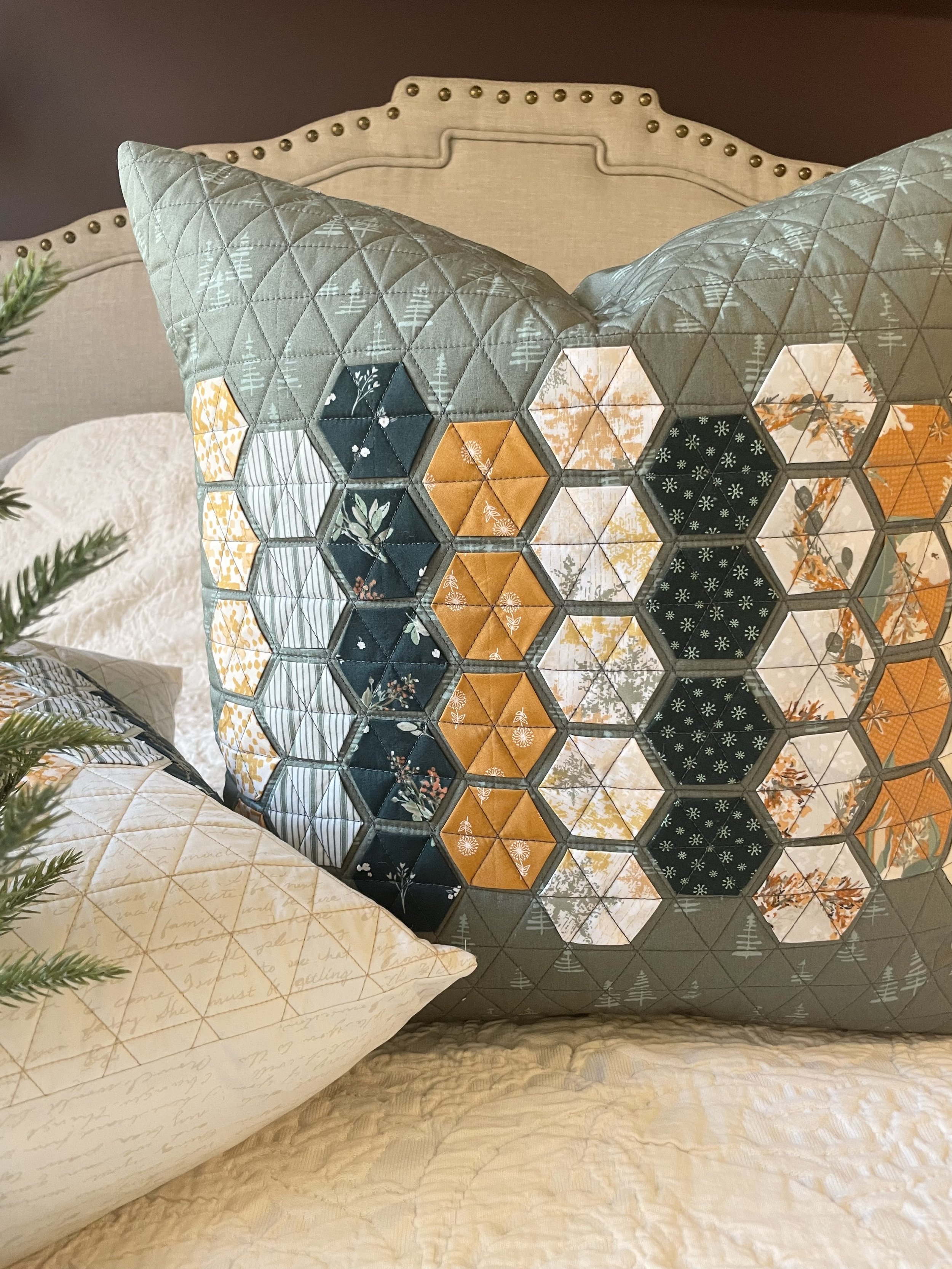This photograph features a stylish bedroom setting centered around a bed with a fabric headboard that boasts a soft, arch design and is adorned with studs along the top. The headboard is off-white, set against a brown wall, adding a subtle yet sophisticated touch to the overall ambiance. The bed is dressed with a creamy quilt blanket that provides a neutral backdrop for the standout pillows.

Dominating the scene is a large, quilted throw pillow prominently positioned in the center. This pillow serves as the main focal point with its textured, gray background that is delicately printed with tiny white pine trees. Central to this pillow are four smaller, octagonal quilt swatches arranged in a stack. These octagons are adorned with a variety of patterns and colors, including gold, white, yellow, black, blue with white snowflakes, tan, and blue with white foliage, each adding a unique, festive touch to the geometric design.

Accompanying the main pillow are two additional decorative pillows. To the left lies a cream-colored pillow with some form of script or writing, providing a simplistic contrast to the intricate design of the main pillow. Another matching pillow, also cream and featuring writing, lies on its side.

Adding an unexpected element to the photograph is a bit of greenery; pine needles or a part of an evergreen tree intrudes slightly from the left, suggesting a seasonal or natural decorative theme. The combination of textures, colors, and patterns creates a cozy and visually appealing arrangement that captures the essence of thoughtful interior décor.